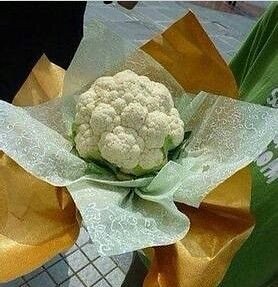The photograph showcases a head of cauliflower, characterized by its numerous sections and fresh green leaves at the bottom, resting on an array of layered wrapping papers. The outermost layer is a light green paper with an ornate design, under which lies a gold paper, and beneath that, a mosaic-patterned surface is visible, possibly part of a countertop or floor. To the left, there appears to be a green shopping bag, while on the right, white tissue paper is draped around it. Additionally, a person wearing a green t-shirt with some indistinguishable white lettering is partially visible, seemingly holding the cauliflower. The scene exudes a fresh and vibrant aesthetic, accentuated by the intricate and colorful wrappings around the cauliflower.